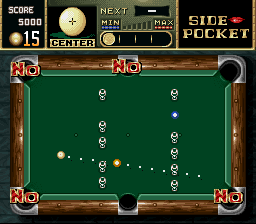In this detailed image, we see the screen of a video game showcasing an overhead view of a pool table. The virtual pool table, covered in green felt, is illuminated with three distinct balls: one blue, one white, and one orange. Prominently displayed in the upper right corner is the text "Side Pocket," while the upper left corner shows the numbers "5,000" and "15." Centered on the screen, the words "Minimum" and "Maximum" appear on the top line. The pool table features the traditional six pockets, with two located at each end and two at the sides. Interestingly, the word "No" is marked on four out of the six pockets, potentially indicating restricted targets. Adding to the complexity of the scene, there is a detailed diagram on the table, illustrated with small white dots, indicating the suggested direction and manner in which to shoot the ball.